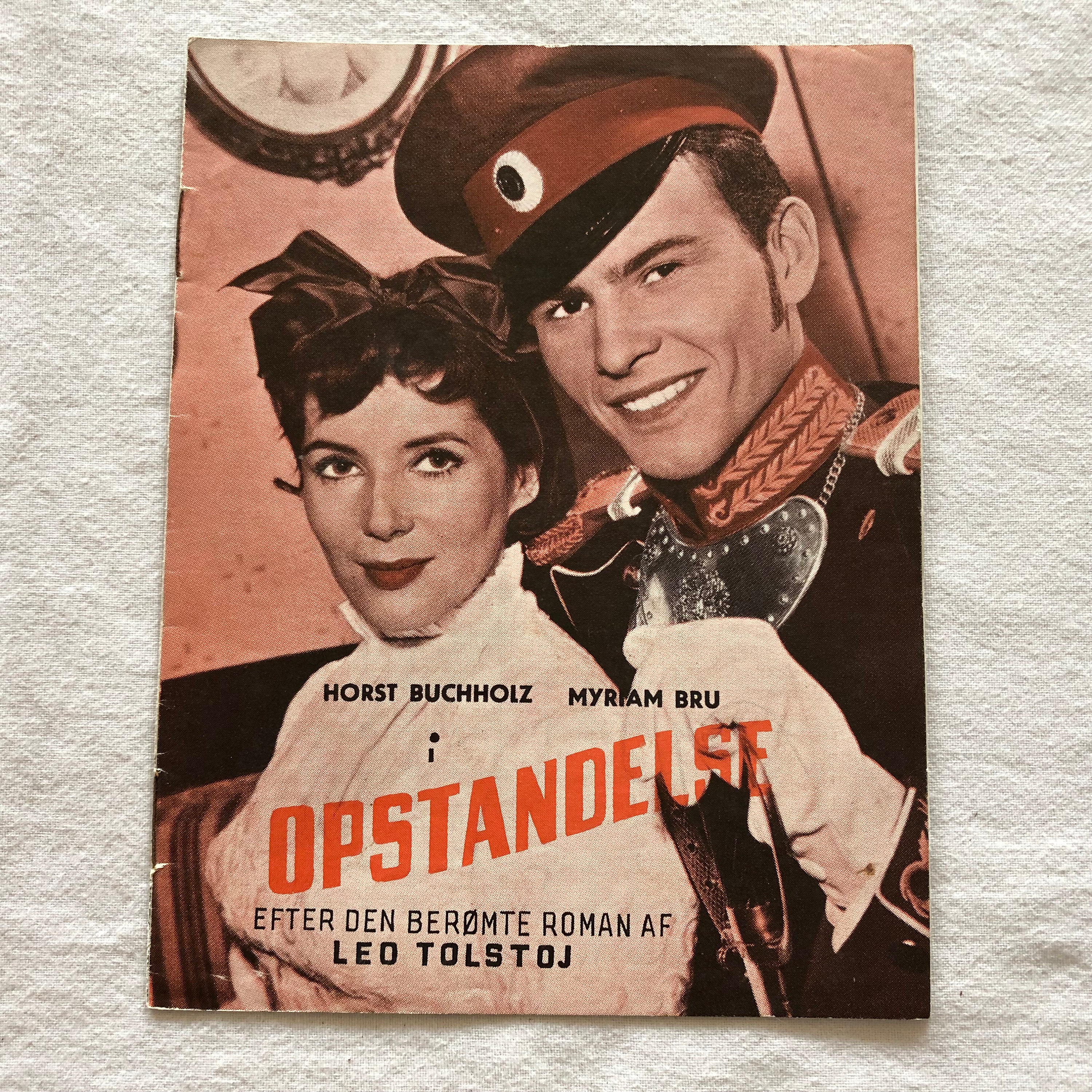In this black-and-white photograph, a distinguished military gentleman and a graceful lady stand side by side, facing the camera. The gentleman is impeccably dressed in a military uniform, featuring a brown army hat and white gloves, and he holds a leather strap in his left hand. He is clean-shaven and exudes a polished, handsome appearance. The lady beside him is equally striking, with short hair neatly styled and adorned with a large bow tied at the top. She wears dark red lipstick that contrasts beautifully with her pristine, white frilly top. Her eyes are soft yet confident as she stands next to the military man. 

The names "Horst Buchholz" and "Myra Mbru" are prominently displayed, though it's unclear whose name belongs to whom. Above them in bold orange letters, the title "Opstandelse" grabs attention, while beneath it, the text "Efter den Veromteroman af Leo Tolstoj" adds an intriguing cinematic or literary context to the scene. The photograph captures both their distinct personalities and the significant era they represent.